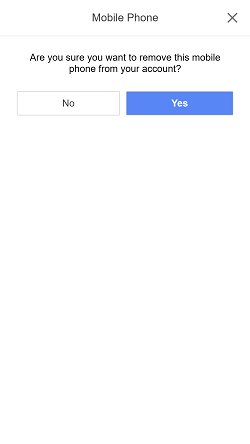The image appears to be a screenshot from a mobile phone, featuring a pop-up dialogue box with a white background. The dialogue box contains a message that reads, "Are you sure you want to remove this mobile phone from your account?" Below the message, there are two options: "No" and "Yes." The "No" option is presented in plain white text, while the "Yes" option is highlighted in blue text, potentially to encourage the user to select it or to indicate it has already been selected. The overall design is minimalist, with standard font and no additional graphical elements, emphasizing the importance of the decision at hand.